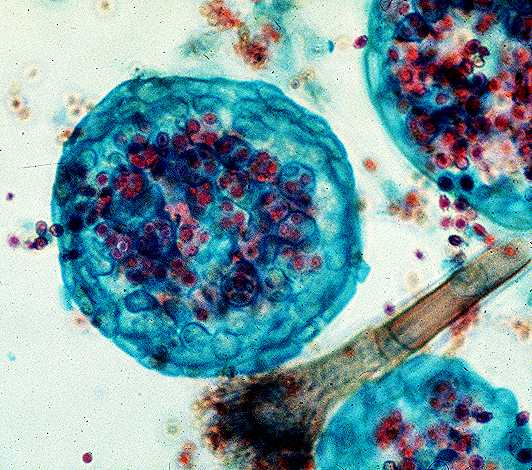This detailed, colored photograph captured through a microscope exhibits a fascinating view of cells, potentially from an animal or a human body. The background is a soft beige, creating a stark contrast to the vibrant scene within. Central to the image are three prominent, circular cells, each a translucent aqua blue, dotted with smaller structures in hues of dark blue, red, purple, and brown. These smaller circles densely populate the larger ones, suggesting cellular components or inclusions. Interspersed among these cells, the background is sprinkled with tiny, colorful flecks in shades of light blue, red, orange, and beige, adding to the textured intricacy of the scene. Diagonally bisecting the composition is an elongated, thin structure, tan beige in color with a darker tip, resembling a delicate bamboo stick or bone fragment. This structure seems to interact with the circular cells, enhancing the enigmatic and complex narrative of the microcosm depicted.